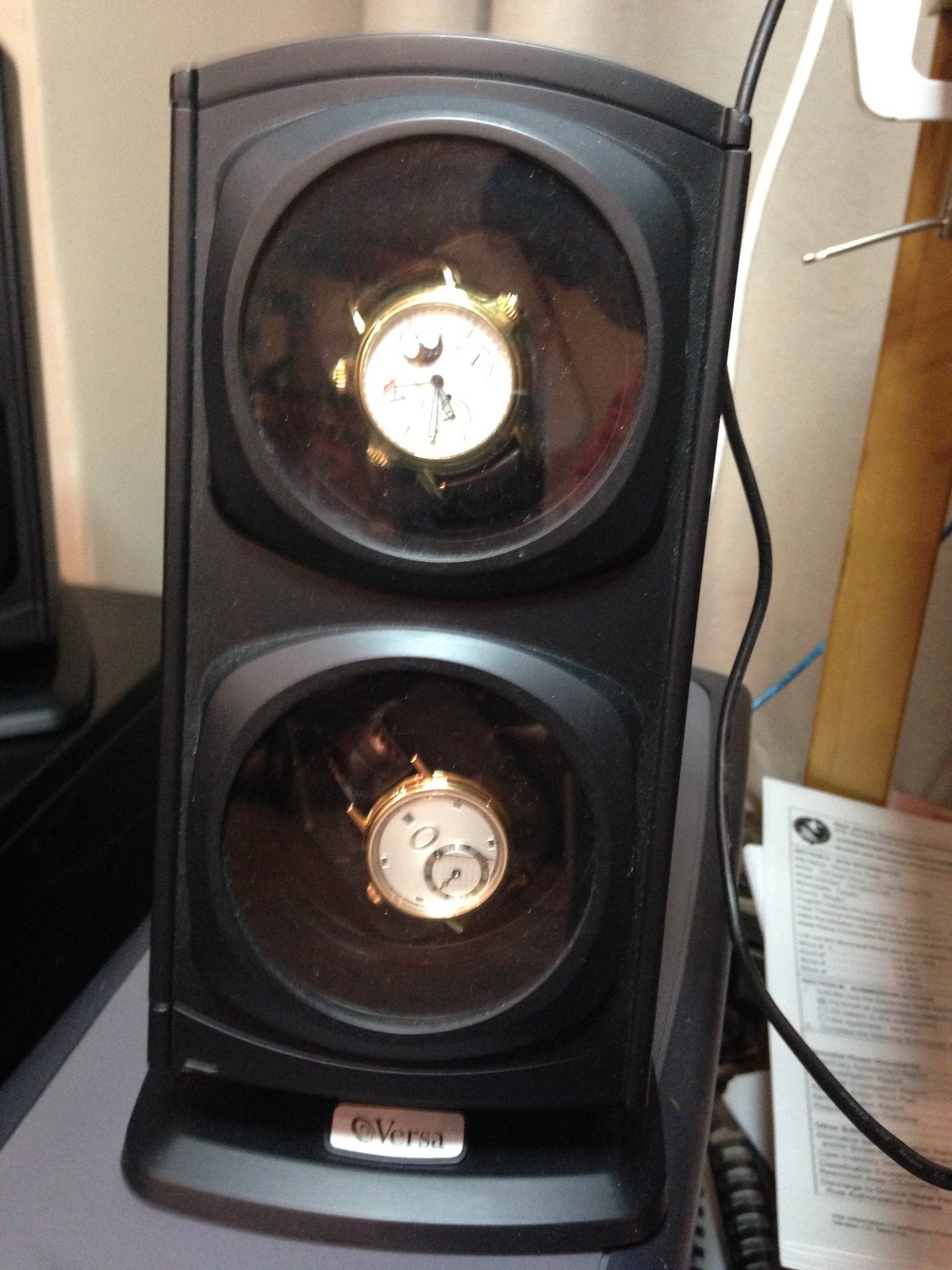This detailed close-up showcases a unique and sophisticated display case designed to hold two luxurious watches, positioned horizontally one above the other. The display bears a slight resemblance to a stoplight and rests elegantly on a desk, encased in a sleek black frame. Each watch is snugly enclosed within its own protective bubble. 

A security cord threads through the hinge of the case, adding an element of safety. The upper watch is a distinguished gold timepiece with a rich brown leather band, likely intended for men. This watch features a moon phase complication on its dial, with prominent, coarse winding crowns.

The lower watch mirrors the top in its luxurious design, also crafted from gold and complementing a thick leather strap. Its dial is adorned with an infinity symbol and a secondary small second-hand sub-dial.

The case bears the brand label "Versa" at its base, signifying the quality and prestige of the items within. Scattered to the right of the image are some miscellaneous clutter including paper and a foam cord, giving the scene a lived-in, authentic atmosphere.